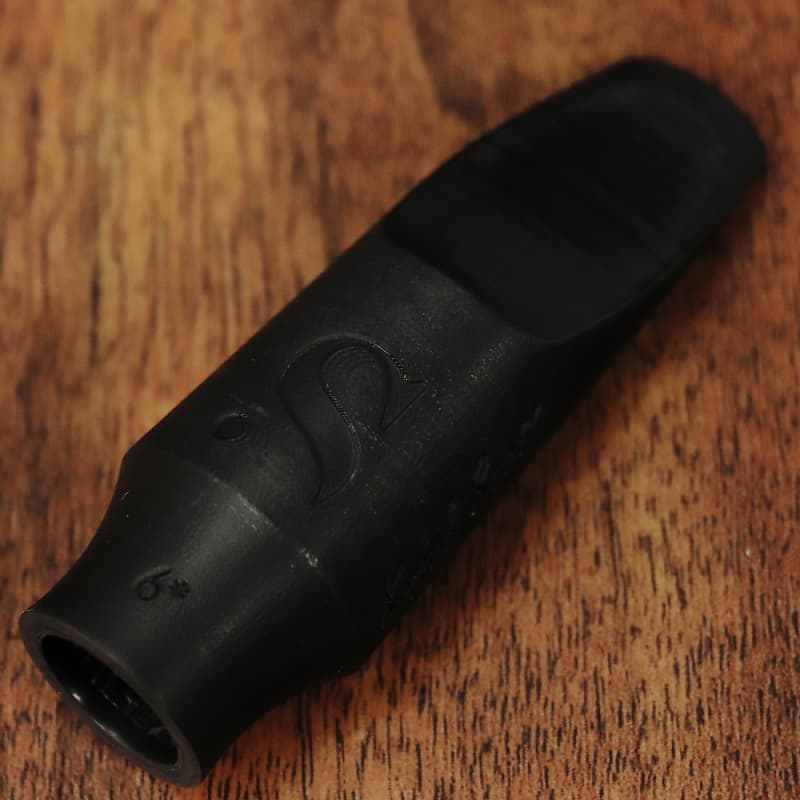This is a close-up photograph, probably taken indoors, of an unidentified black, cylindrical object with a distinctive shape. The object, which might be made of rubber or metal, begins with a narrow cylinder that broadens into a larger, rounded end. This larger section has an opening facing toward the bottom left corner of the image, while the rounded tip points toward the top right. Notably, there is a number nine carved into the side of the device. The object resembles an attachment, possibly for a vacuum, or another kind of appliance, and is lying on what appears to be a brown, wooden surface with small black marks. The photograph does not contain any text, making it difficult to discern the precise function or use of the object.